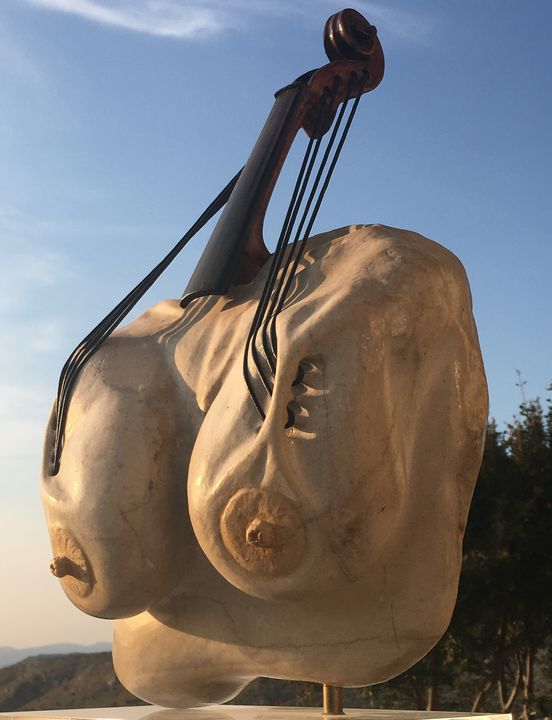The image depicts a striking piece of modern art featuring a surreal sculpture that merges elements of a woman's torso with a musical instrument, likely a cello or violin. The central focus is on the exaggerated, sagging breasts, with pronounced nipples, which dominate the composition. The sculpture is devoid of a head and arms, further emphasizing the breasts as the main subject. Emerging from where the neck would typically be is the top part of a violin or cello, with strings extending outward and appearing to dig into the sides of the breasts, almost as if they are functioning as hands. The setting is outdoors, under a light blue sky with some clouds, accompanied by the dark silhouettes of trees in the background. This unusual and provocative piece of artwork elicits a sense of unease with its use of anatomical and musical elements combined in a way that challenges traditional perceptions.